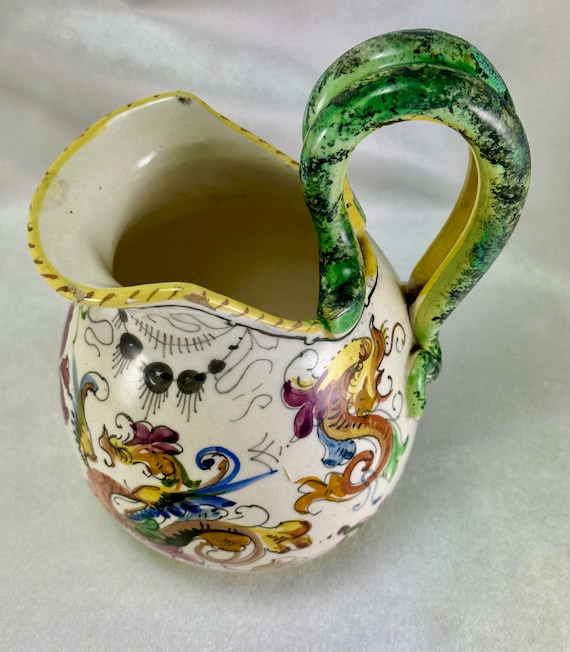Photograph Description: A detailed ceramic vase showcases an intriguing blend of artistic elements. The vase is predominantly white, constructed from high-quality ceramic or clay, with a glossy, creamy interior. A lime green, organically shaped handle arches gracefully from its side, resembling twin snakes juxtaposed. This handle features a delicate speckled black pattern and is accentuated with a subtle yellow trim.

The vase’s mouth curves forward elegantly, culminating in a broad lip at the front, which is also adorned with a yellow trim adorned with beige hash marks. The body of the vase is richly decorated with intricate illustrations, including depictions of brown and yellow fish. Interspersed among these aquatic motifs are black and white patterns, harmoniously integrated into the overall design.

The background of the image is a soft, whitish cloth, providing a neutral and minimalist backdrop that enhances the details and textures of the vase. The combination of colors and patterns on this unique piece reflects both artistic creativity and meticulous craftsmanship.